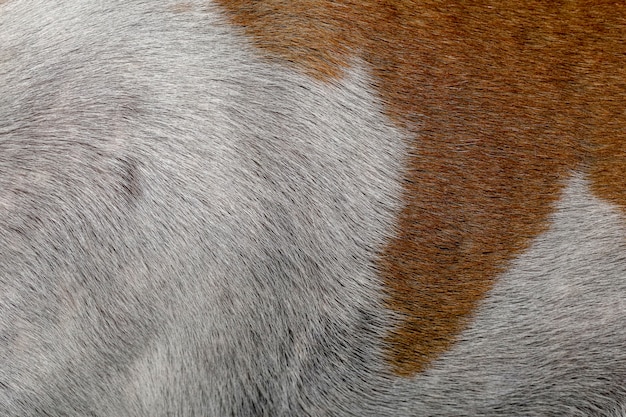This is a rectangular, close-up photograph of an indeterminate animal, showcasing a side view that includes a prominent fur pattern. The majority of the image is dominated by thick, white fur overlaying dark, almost black skin. This fur is characterized by minor variations but remains predominantly white, with the skin occasionally peeking through. A significant asymmetrical, light brown or burnt orange patch swoops down from the top right corner, resembling a large finger or thumb extending almost to the bottom of the frame. The animal's side is slightly contoured, possibly hinting at the shoulder or hip area, yet lacks definitive features to identify the species. The fur appears short-haired, and the overall close-up composition makes it challenging to discern whether this is a dog, cow, horse, pig, or another mammal.